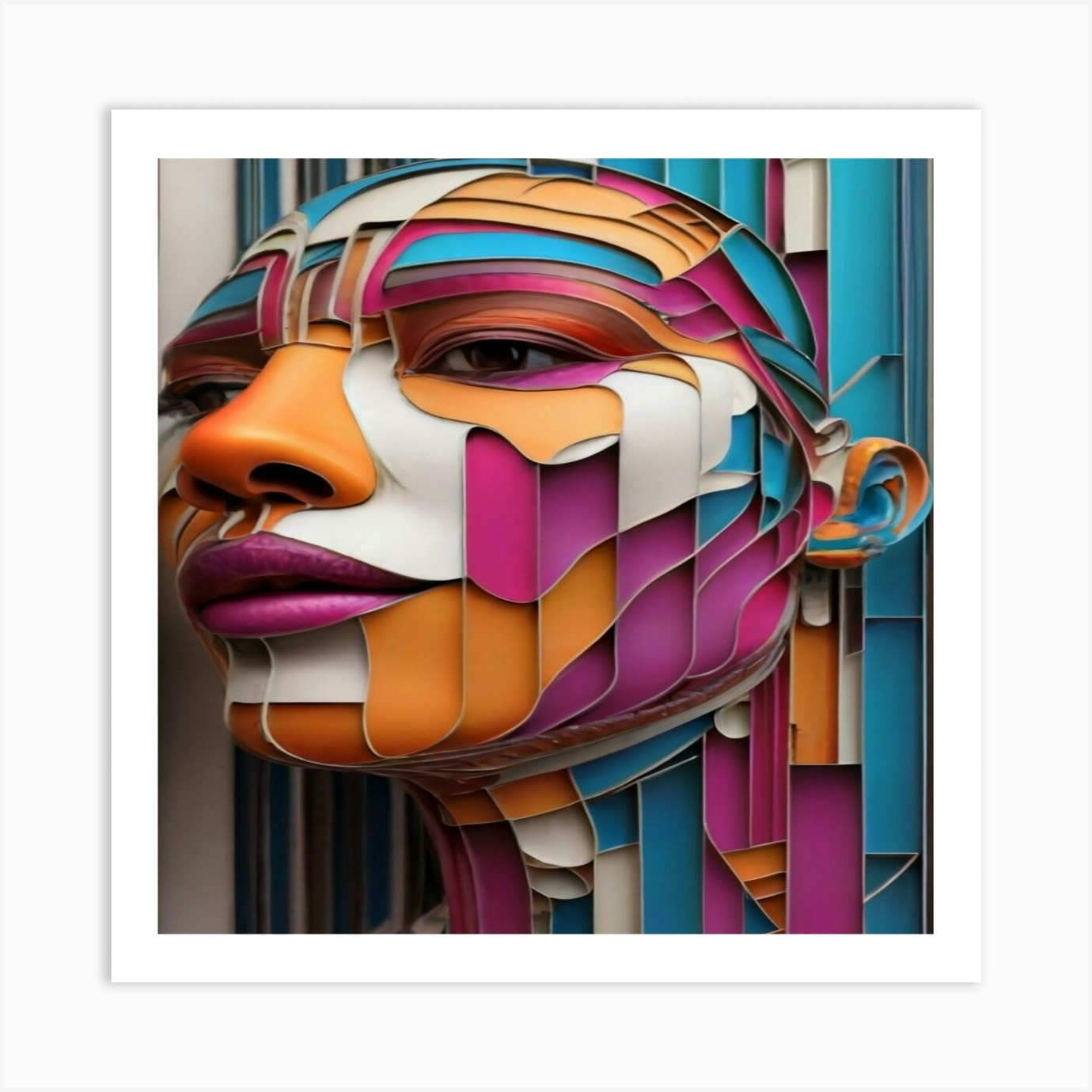This image displays a square artwork, approximately six inches in height and width, set against a plain light gray background. The artwork itself is bordered by a white frame about a quarter to half an inch wide. Inside this frame is a smaller square, around four inches high and wide, which features a vibrant and abstract depiction of a woman's face looking to the left. The face is composed of numerous rectangular and curved panels, each populated by distinct colors such as blue, violet, white, orange, teal, tan, light brown, light purple, and dark purple. These panels are outlined with raised white edges, adding a three-dimensional effect to the artwork. The woman's face showcases lifelike features including white and brown eyes, an orange nose, pink and purple lips—dark purple on the upper lip and light purple on the lower lip—and various panels in shades of blue, pink, white, and purple across her cheeks and forehead. These meticulously delineated shapes converge to form a cohesive and dynamic portrait.